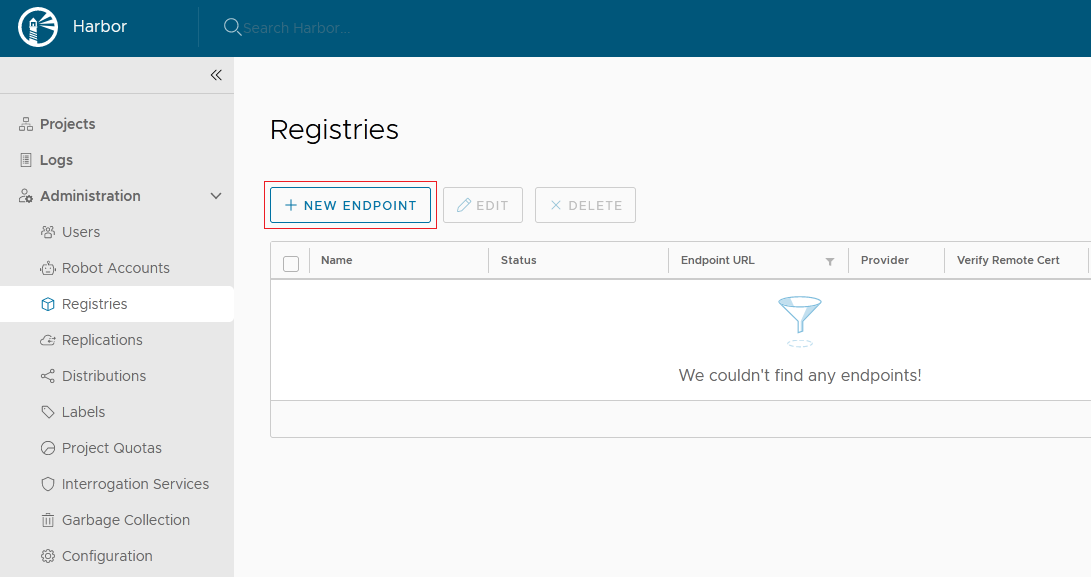Here is a cleaned-up and detailed caption for the image:

---

This image is a screenshot of a user interface for a website with a predominantly pale grey color scheme. The navigation bar on the left side of the screen is a slightly darker grey, while the top bar is a deep teal color. In the top left corner of the teal bar, there is a white lighthouse logo encircled by the word "Harbour" in white, with the search bar featuring a magnifying glass icon next to it.

The navigation bar below the "Harbour" header lists various options in white text on the darker grey background. These options include: Projects, Logs, Administrator, with expanded sub-options under Administrator, such as Users, Robot Account, Registries, Duplications, Distributions, Labels, Project Quotas, Interrogation Services, Garbage Collection, and Configuration.

The user is currently on the "Registries" tab, which opens a main panel to the right, occupying the majority of the screen. At the top of this main panel, the heading "Registries" appears in black text against a light grey background. Below this, there is a section highlighted by a red rectangle around the "New Endpoint" button. Beneath this button, a results section reads, "We couldn't find any endpoints," indicating that no registry endpoints are currently available.